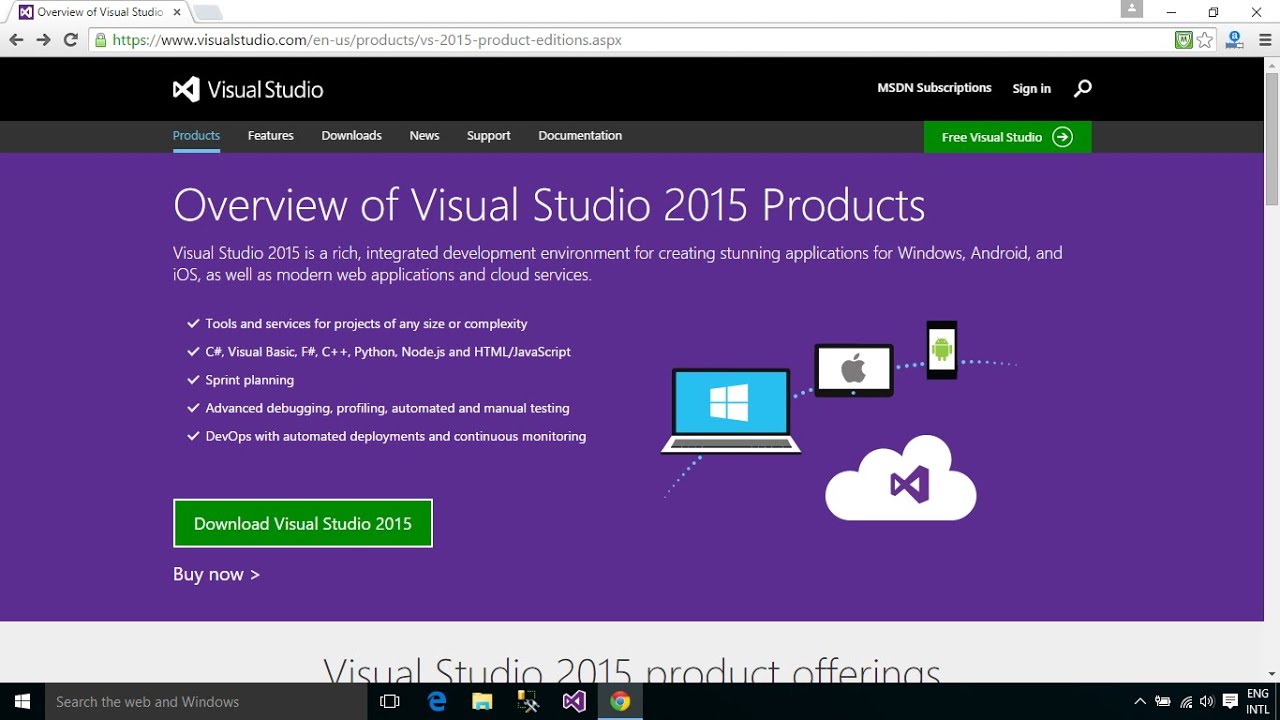**Caption:**
"An in-depth overview of Visual Studio 2015 is presented on the official Visual Studio website at visualstudio.com. Visual Studio 2015 serves as a comprehensive integrated development environment (IDE) designed for creating applications across various platforms, including Windows, Android, and iOS. It also supports the development of modern applications and cloud services, offering tools and services suitable for projects of any size or complexity. The environment supports multiple programming languages such as C#, Visual Basic, F#, C++, Python, Node.js, and HTML/JavaScript. The website's layout features a black background with a central visual element consisting of a laptop displaying the Windows logo, a tablet showing the Apple logo, and a phone featuring the Android logo. Below these devices is the emblematic logo of Visual Studio 2015, which can be interpreted in various ways."